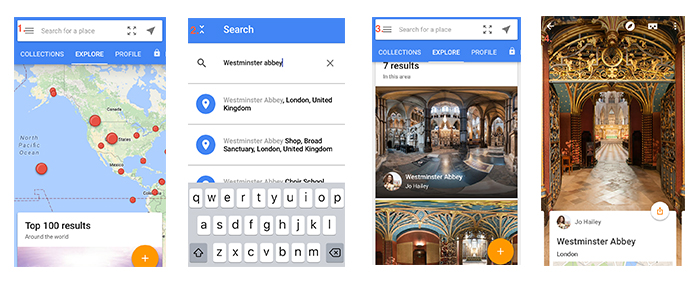This image comprises four distinct screenshots from a person's phone display, each showcasing a different section. Here’s a detailed descriptive caption for the image:

The composite image comprises four screenshots taken from a mobile phone, each providing a unique visual and informational perspective related to global search results and Westminster Abbey. The first screenshot on the left features a world map labeled "Top 100 Results Around the World," scattered with red dots of varying sizes pinpointing notable locations, prominently highlighting areas in the United States, Alaska, the Panama Canal, and extending into South America. The second screenshot reveals a search interface with the query "Westminster Abbey," displaying two results: "Westminster Abbey, London, United Kingdom," and "Westminster Abbey Shop, Broad Sanctuary, London, United Kingdom," accompanied by an active on-screen keyboard. The third image shows seven search results with a detailed interior view of Westminster Abbey, capturing its intricate ceiling, ornate lighting, and an orange plus sign at the bottom for additional options. The fourth and final screenshot presents an exterior view of Westminster Abbey in London, encapsulating its iconic architectural façade.